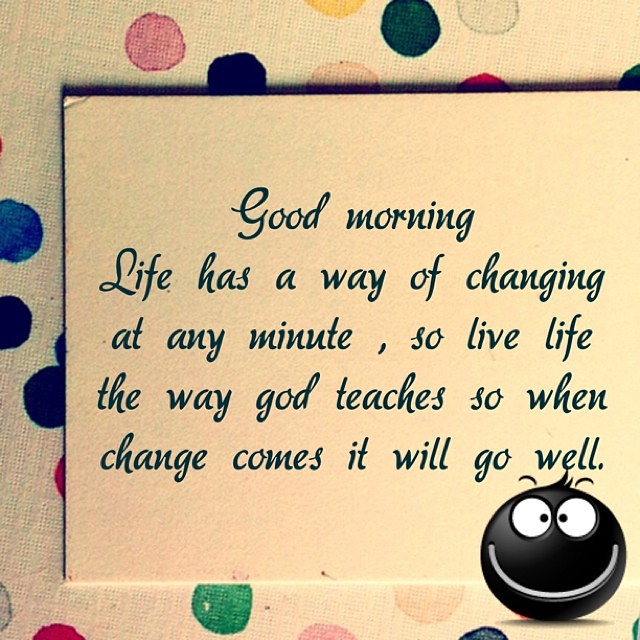The image depicts a framed or poster-like message with a motivational quote. The background is light yellow or off-white, with elegantly scripted black text that reads, "Good morning. Life has a way of changing at any minute, so live life the way God teaches. So when change comes, it will go well." The message is presented on a thick, rectangular board. In the bottom right corner, there's a whimsical character—a green, circular smiley face with white eyes and black pupils, sporting a wide smile. This character adds a playful touch to the scene. The background surface is covered with a polka-dotted pattern in a variety of colors, including pink, green, white, red, off-white, purple, blue, and magenta, and resembles fabric with visible threads, giving the image a textured look.